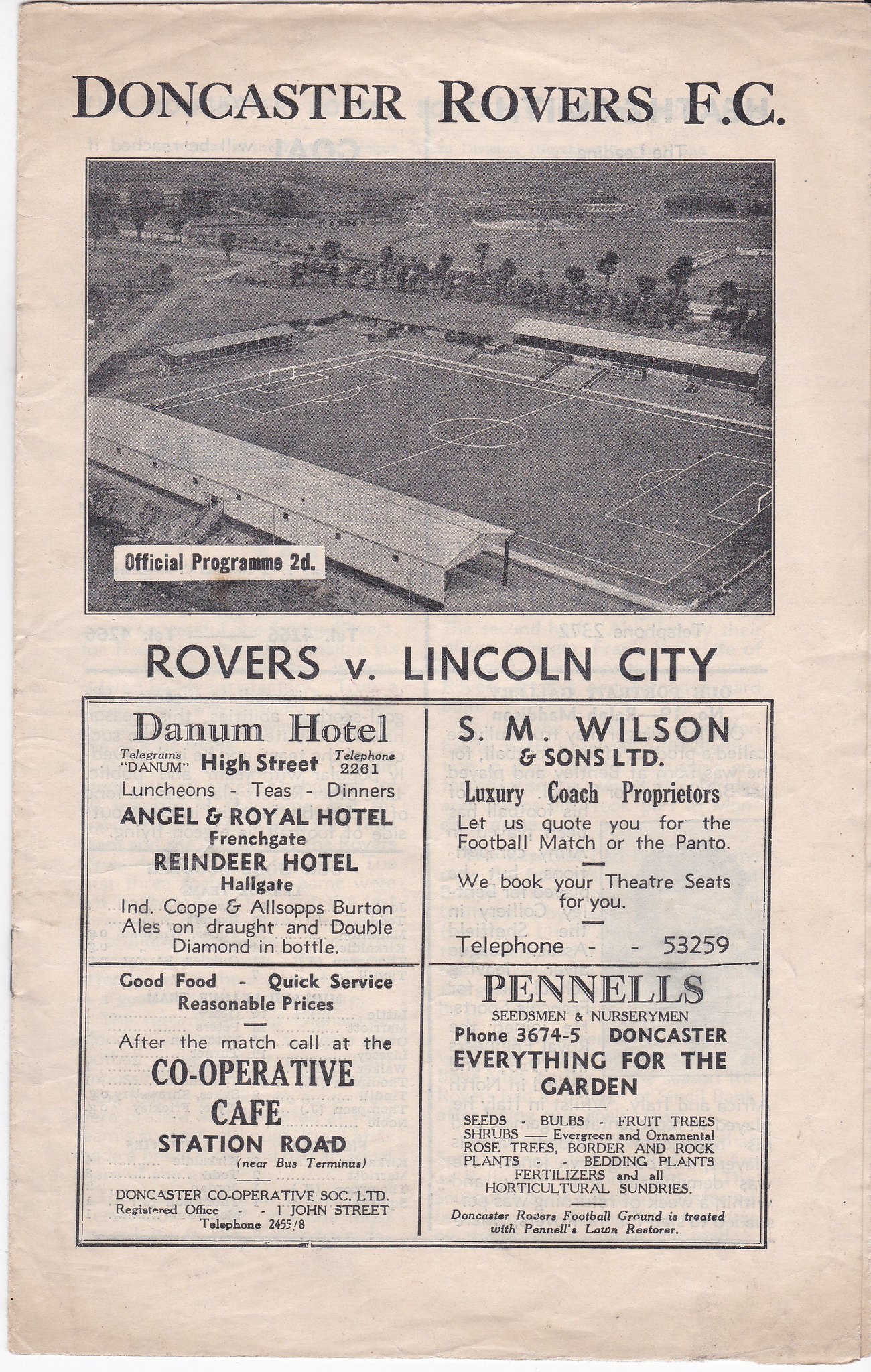This image depicts an aged, possibly worn-out official program from a soccer match, featuring a faded black and white photograph at the top. The large title "Doncaster Rovers FC" is prominently displayed, with an aerial view of a soccer field below it. The field includes goal posts at each end, painted markings, and surrounding bleachers, with trees and additional sports fields visible in the background. On the left, there's a header "official program 2D" next to the field photo. Below the field, the text "Rovers v Lincoln City" is present, followed by notable advertisements in four individual squares. These ads include details for Danum Hotel (mentioning High Street, luncheons, teas, and dinners), Angel and Royal Hotel, French Gate, Reindeer Hotel, and additional businesses like S.M. Wilson and Sons LTD (specializing in luxury coach services), Cooperative Cafe (promoting good food, quick service, and reasonable prices), and Pinnell's Doncaster (offering gardening supplies). The advertisement for Wilson and Sons also offers theater seat bookings, suggesting a historical community focus.